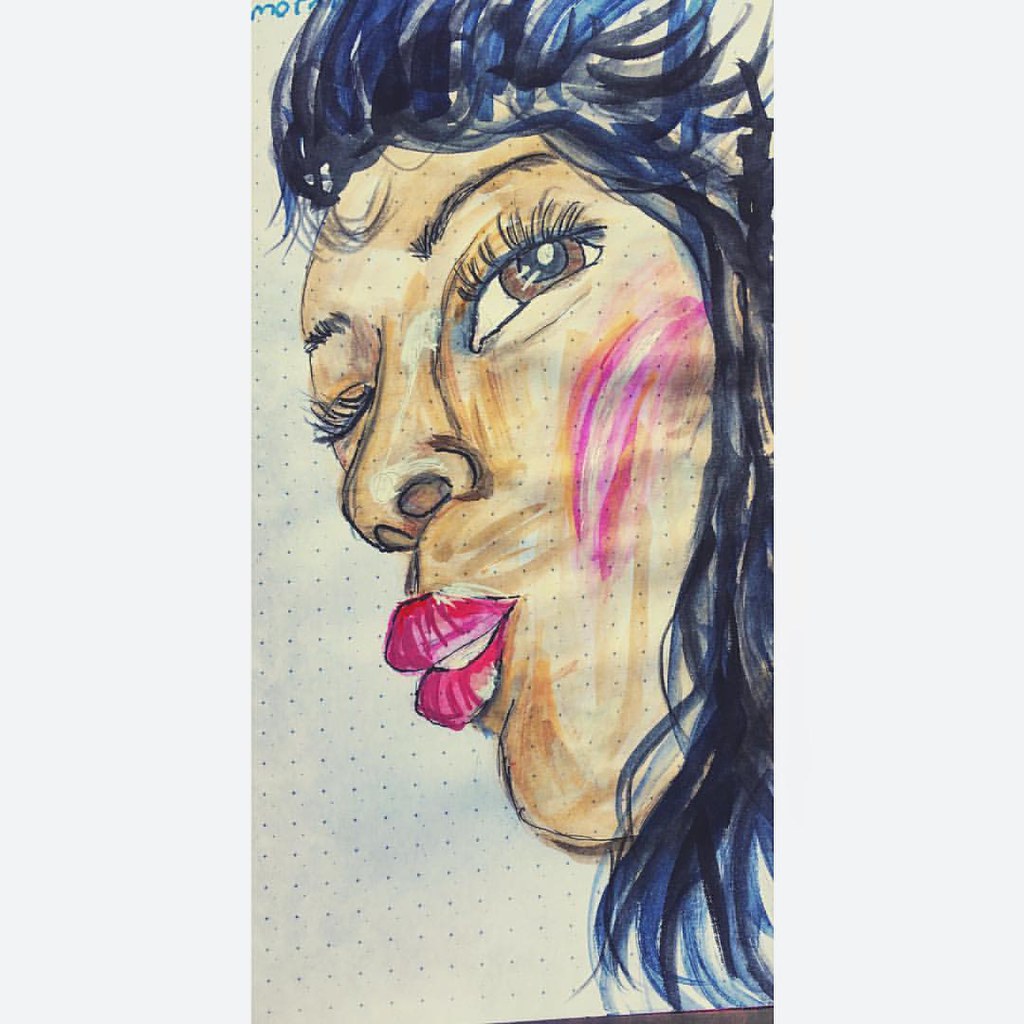The image is a rectangular drawing, potentially done with markers, chalk, or colored pencils, depicting a stylized black woman against a background of evenly spaced black polka dots. Her striking black hair, accentuated with hints of blue, is styled high and cascades down over her left shoulder, partially covering that side of her face. She has distinct facial features, including a large, open brown left eye with long eyelashes, well-groomed black eyebrows, and a closed right eye giving the impression of a playful wink. Her skin has a dark complexion, accentuated with blush that creates a pink, red, and white gradient on her cheekbones, adding dimension to her face. Her full, vivid red lips are slightly parted, revealing a bit of her teeth in a subtle smile. The composition focuses solely on her head, without showing her neck or shoulders. The piece is signed at the top left, where the letters "M.O." and possibly more are visible in blue. The overall effect is a vibrant, detailed depiction of the woman's expressive face against the minimalist, polka-dotted backdrop.